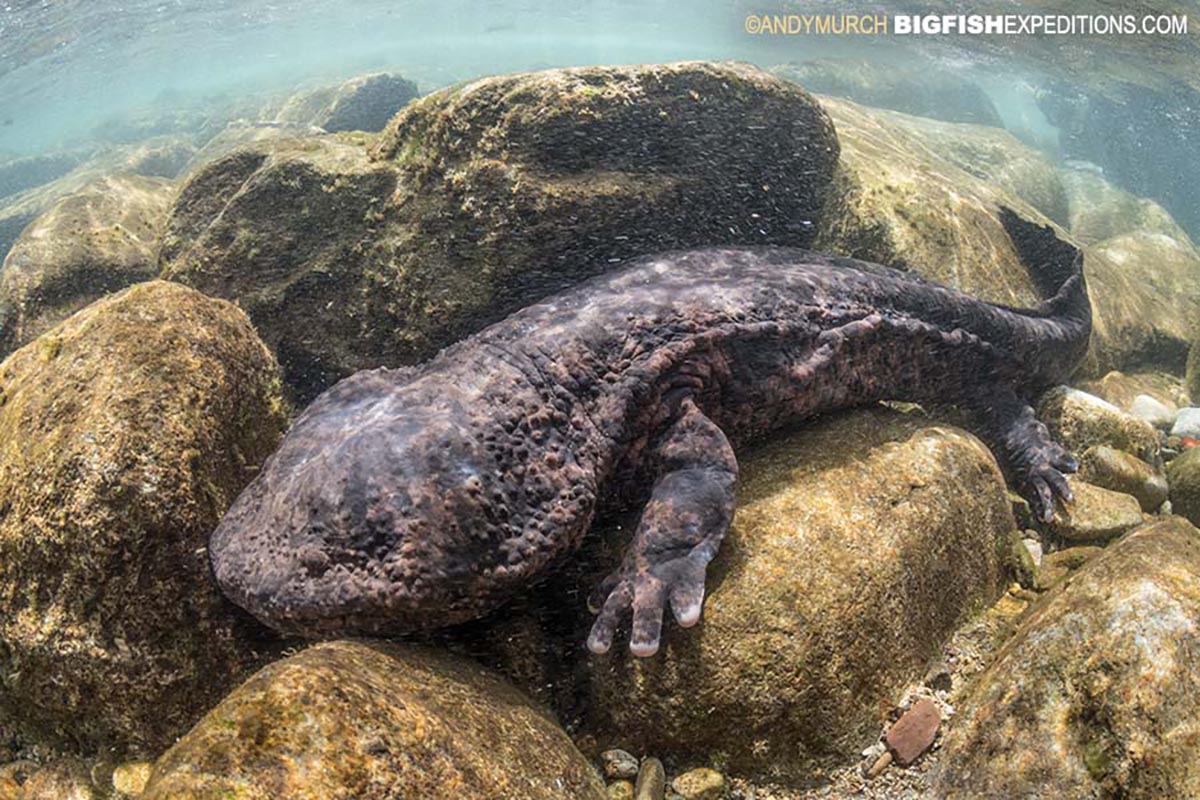This underwater photograph, a horizontal rectangle about 1.5 to 1.75 times as wide as it is tall, captures a large dark-colored lizard, potentially a Gila monster, lying on a rocky ground composed of large black, brown, and beige rocks. The lizard, with its broad head and elongated body displaying shades of dark brown, black, and hints of dark purple, has four legs with stubby fingers, one leg resting on a rock in the front and another hanging off in the back. The water above is a murky blend of bluish-green with a strip of light blue-gray at the top. In the upper right-hand corner, white and orange text reads "© Andy Murich, bigfishexpeditions.com."